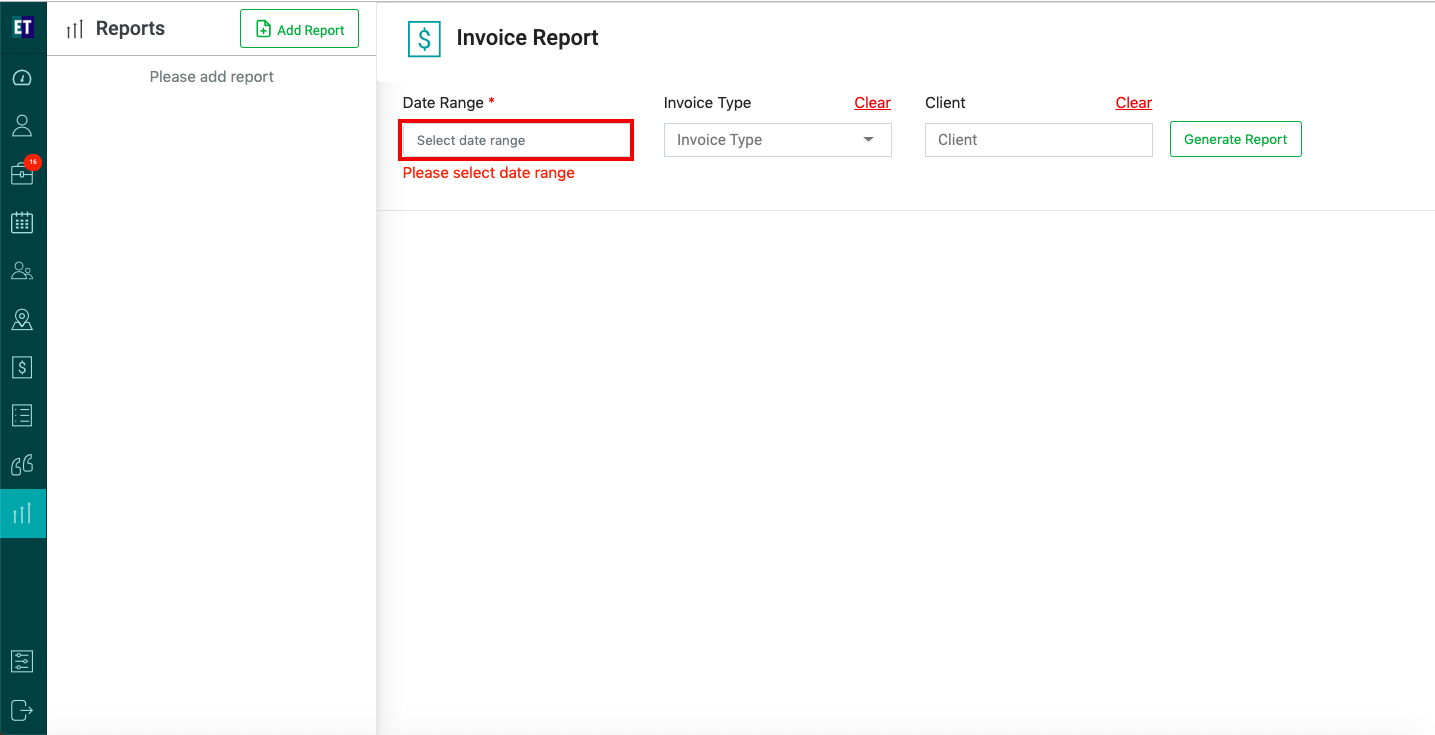The screenshot depicts a financial or accounting software interface. On the far left, there is a very thin menu bar with at least 10 icons. The currently highlighted icon resembles a bar graph with three vertical lines increasing in height. This icon corresponds to the "Reports" tab. 

In the central section, there's a button labeled "Add Report." 

The rightmost panel is titled "Invoice Report." At the top of this panel, "Date Range" is highlighted in red. A text box below it prompts the user to "Select Date Range," and beneath this box, the text "Please select date range" is displayed in red, indicating an error or mandatory action. 

Next to the date range selector, there is a dropdown menu for "Invoice Type," followed by a text box for entering the "Client's Name." At the bottom of this panel, there's a button labeled "Generate Report."

The interface appears to be designed for generating and managing various financial reports, with user prompts to ensure the correct input of information.